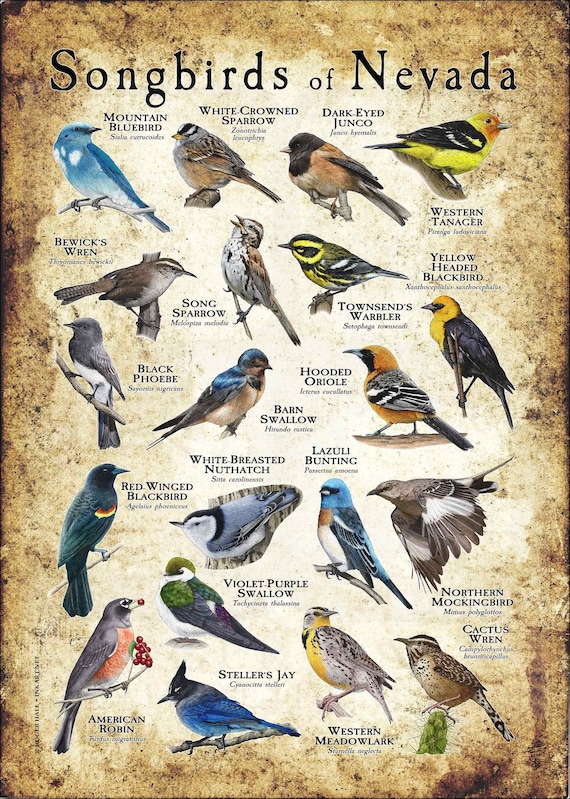The image is a detailed, full-color poster titled "Songbirds of Nevada," presented in black text at the very top. The poster is vertically rectangular and appears to be a scan of an artistic representation, not photographs, of various bird species. The background transitions from brown on the edges to a cream color in the center. Each bird is illustrated with meticulous detail, and both the English and Latin names are provided in black text.

The top row features the Mountain Bluebird, perched on a tree branch to the left, followed by the White-crowned Sparrow with its distinct white crown. Next are the Dark-eyed Junco, which has brown and black plumage, and the Western Tanager, showcasing bright yellow and black coloring. 

In descending order, the second row starts with Bewick's Wren on the left, followed by the Song Sparrow, Townsend's Warbler, the Black Phoebe, the Barn Swallow, and the Hooded Oriole, extending to the far right with the Yellow-headed Blackbird.

The third row includes the Red-winged Blackbird with its striking red and yellow markings, the White-breasted Nuthatch, the Lazuli Bunting sporting blue and white with a touch of brown, and the Northern Mockingbird.

On the bottom row, we find the American Robin, noticeable for its gray body and pink chest, accompanied by the Violet-purple Swallow with a green head, the Steller's Jay, which is blue with a black head, and the Western Meadowlark. Finally, the Cactus Wren is positioned at the far-right bottom.

The poster features around 15 to 20 bird illustrations, making it an intricate and educational display of Nevada’s diverse songbird population.